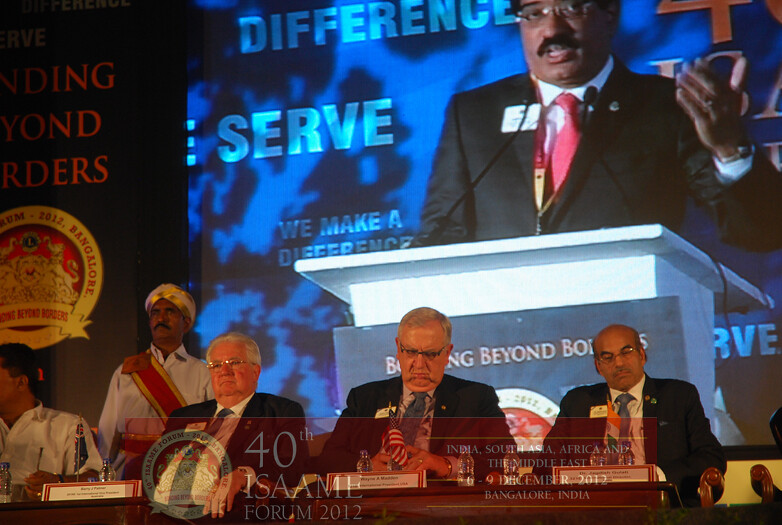In this image, several men are seated at a long table, each with a name card and a small country flag in front of them. The three men at the center draw the most attention: On the left is an older, white man with short gray hair and glasses, wearing a blue suit, white shirt, and blue tie, looking slightly to the left. In the middle sits another older white man, also with short gray hair and glasses, clad in a dark suit, white shirt, and blue tie, looking down and forward. To his right, we see a man with a dark suit, white shirt, and light blue tie; he has a bald top head with black hair on the sides and is looking down and to the right. To their left, partially out of the image frame, is an individual with black hair wearing a white shirt, whose attire differs from the central figures.

In the background, a man stands with a red sash across his chest and a black mustache, wearing a white shirt, looking forward. The backdrop features a large screen projecting a man standing at a white podium, dressed in a black suit, white shirt, and red tie. The background of the screen is predominantly blue with various words scattered across, including "40th AMI ISAA Forum 2012," "India,” "South Asia," "Africa," and "Middle East." The event is dated December 9, 2012, in Bangalore, India. The visible words on the podium include "beyond" and a partially readable banner at the top stating "Difference and Serve."